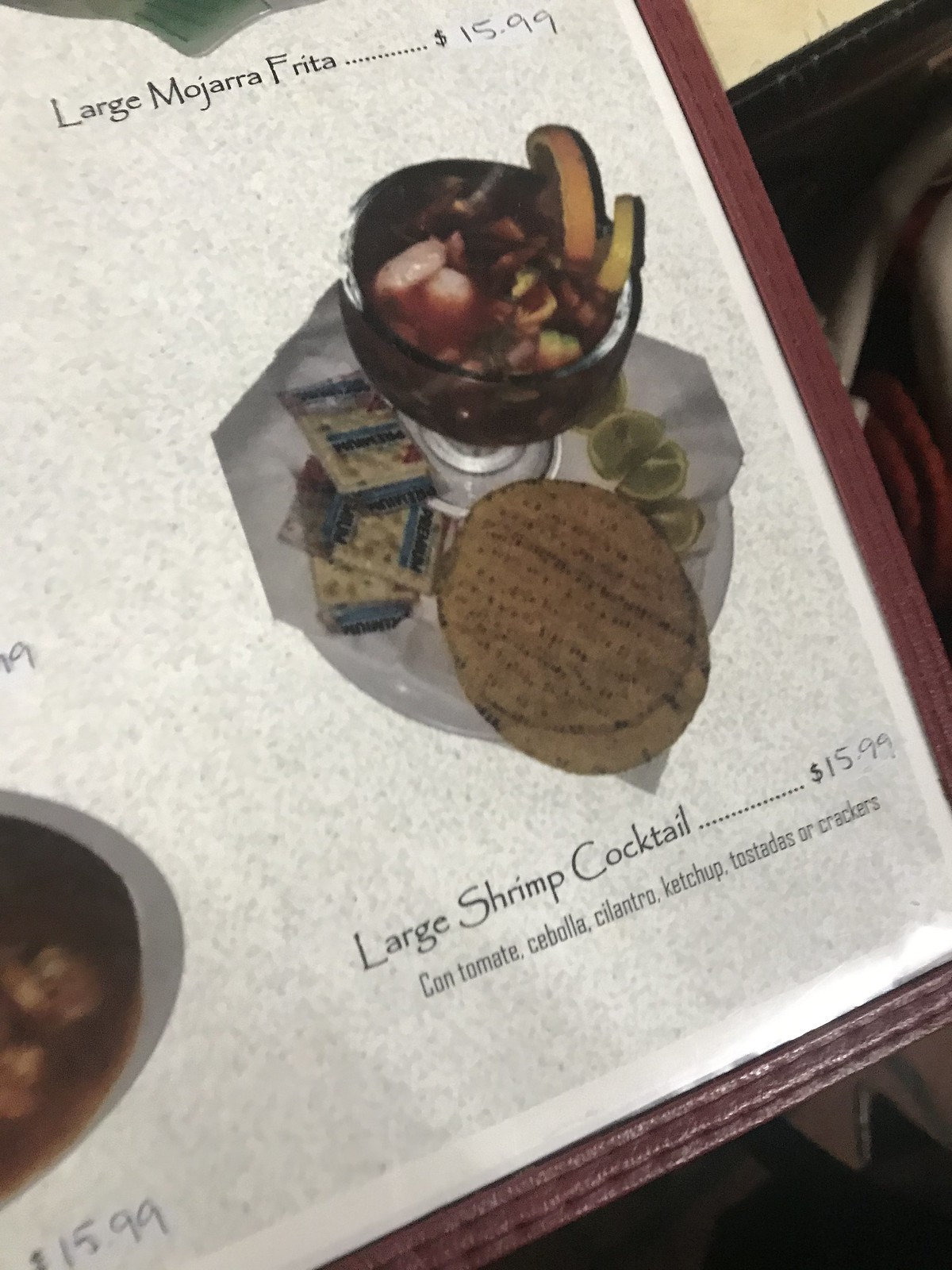A detailed view of a restaurant menu corner is showcased, featuring a red leather rim and a white marbled gradient background. The menu, mostly hanging off the table's black edge with a white interior, highlights a large shrimp cocktail priced at $15.99. This cocktail comes with ingredients such as tomatoes, onions, cilantro, ketchup, and your choice of tostadas or crackers. An accompanying image on the menu depicts the shrimp cocktail, centrally placed with crackers on the side, garnished with the aforementioned ingredients.

Additionally, two other menu items partially appear in the image. One is a large "mojara frita" priced at $15.99, although the image is cut off. Another menu option is visible at the bottom left, showing a price point of $15.99, but the item itself is not fully in the frame. Above it, only the "$99" part of another product's price can be seen, with the rest obscured. The menu's photographic elements look oddly edited, suggesting a rough photoshop job.